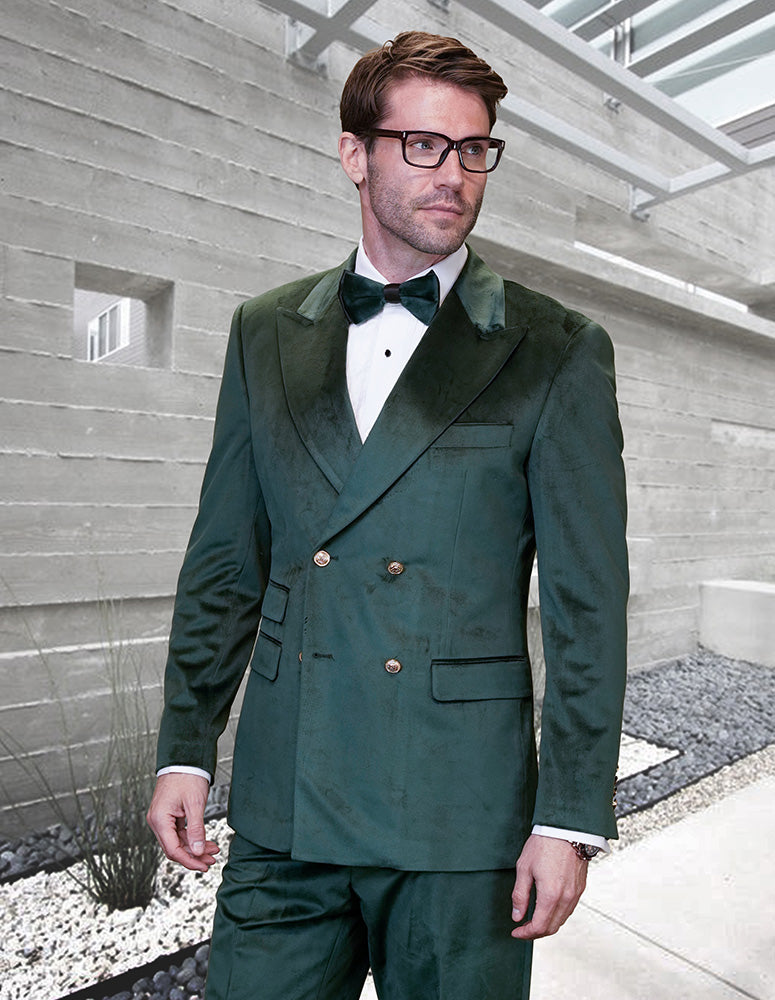In this detailed outdoor photoshoot, a man models a striking green tuxedo ensemble, consisting of a green suit jacket adorned with four buttons, green pants, and a matching green bow tie paired with a crisp white collared shirt. The sartorial elegance is rounded out by black-framed glasses that complement his short, wavy brown hair. He stands posed, with his body angled slightly to the left, while his head is turned contemplatively to the right, providing a thoughtful side profile. This artistic composition is set against a backdrop of a cement brick wall, flanked by a meticulous sidewalk. The ground between the wall and the sidewalk is thoughtfully designed with layers of white rocks interspersed with small, emerging plants, creating an aesthetically pleasing and modern environment.